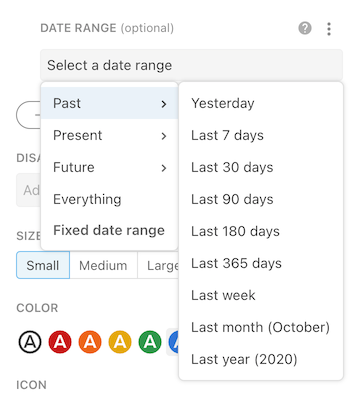The image features a user interface on a white background.

At the top, in all capital gray font, it reads "DATE RANGE" with the word "optional" in lowercase letters enclosed in parentheses. To the right of this text, there is a gray circle containing a white question mark, alongside three vertical gray dots.

Beneath this horizontal section, there is a light gray rectangle with the black text "Select a date range." Below this rectangle, two vertical menus appear, though it's ambiguous whether they are extending from this section or originating from another area.

The first vertical menu features a white background with the following options listed:

- Past (highlighted in light blue with a right-pointing indicator)
- Present (with a right-pointing indicator)
- Future (with a right-pointing indicator)
- Everything (no indicator)
- Fixed Date Range (no indicator)

Adjacent to this, a second vertical menu also on a white background appears, detailing more specific time range options corresponding to the selected "Past" category:

- Yesterday
- Last 7 Days
- Last 30 Days
- Last 90 Days
- Last 180 Days
- Last 365 Days
- Last Week
- Last Month (with "October" in parentheses)
- Last Year (with "2020" in parentheses)

At the bottom of the image, partially obscured by the open menus, there are additional interface elements:

- A "Size" section in gray lettering, offering options of "Small," "Medium," and "Large," with "Small" shaded in light blue.
- A "Color" section in capital light gray font, displaying a sequence of colored options. The first is a black "A" in a white circle with a black outline. The subsequent options feature a white "A" on colored backgrounds: red, orange, yellow, green. Only half of the blue option is visible.
- An "Icon" section in all capital gray font is partially visible below the color options.

This comprehensive layout allows users to select and customize date ranges and visual properties seamlessly.